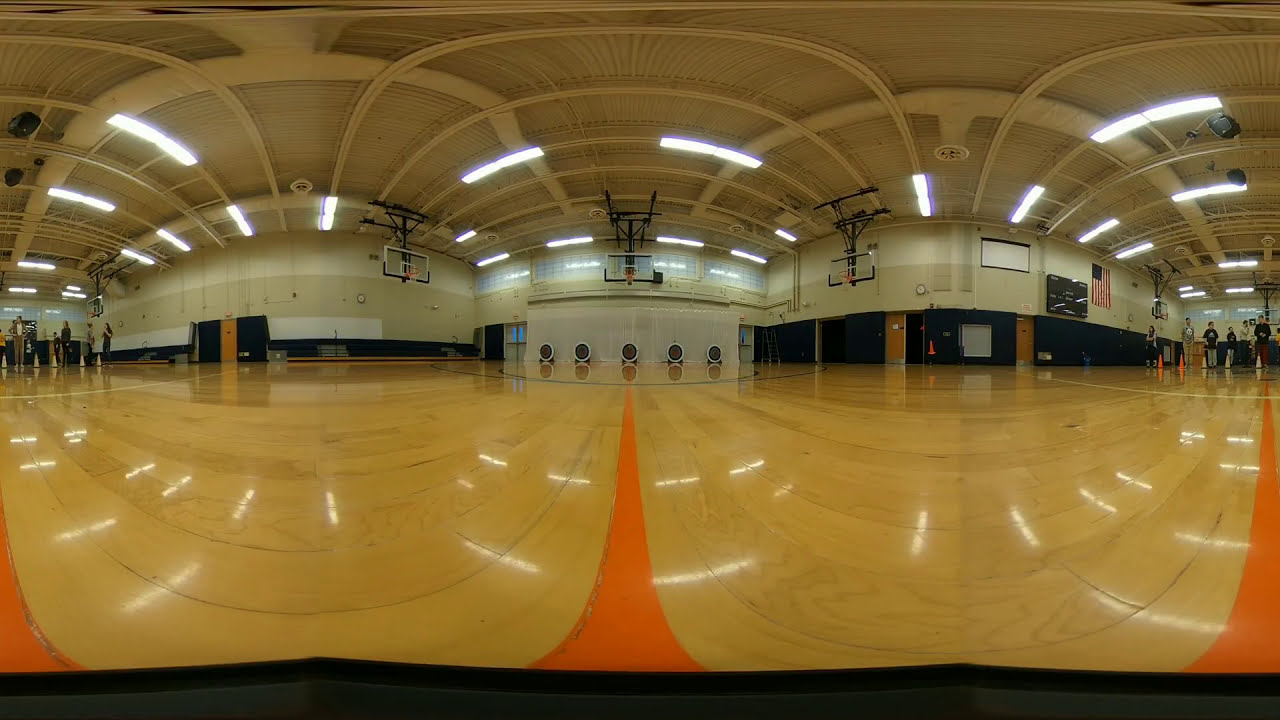This is a panoramic, possibly a 360-degree fish-eye photo of a gymnasium with a glossy, light wooden floor and a white metal ceiling adorned with visible pipes, bars, and beams. The gym is illuminated by numerous fluorescent lights, creating a bright and shiny atmosphere. The walls are painted in a gradient with dark navy blue at the bottom, tan in the middle, and white at the top. Mounted to the ceiling are several basketball hoops, at least three are visible, although the panoramic effect may be multiplying their appearance. 

At the far center of the image, directly underneath what appears to be the main basketball net, are five circular targets resembling archery targets. Running along the left and right sides of the image are lines marked with orange and white cones. Positioned behind these cones are several people, five on each side, lined up as if preparing to engage in an activity, potentially archery given the setup. The skewed and mirrored nature of the photo suggests a duplication effect, giving the impression of an elongated and doubled space.